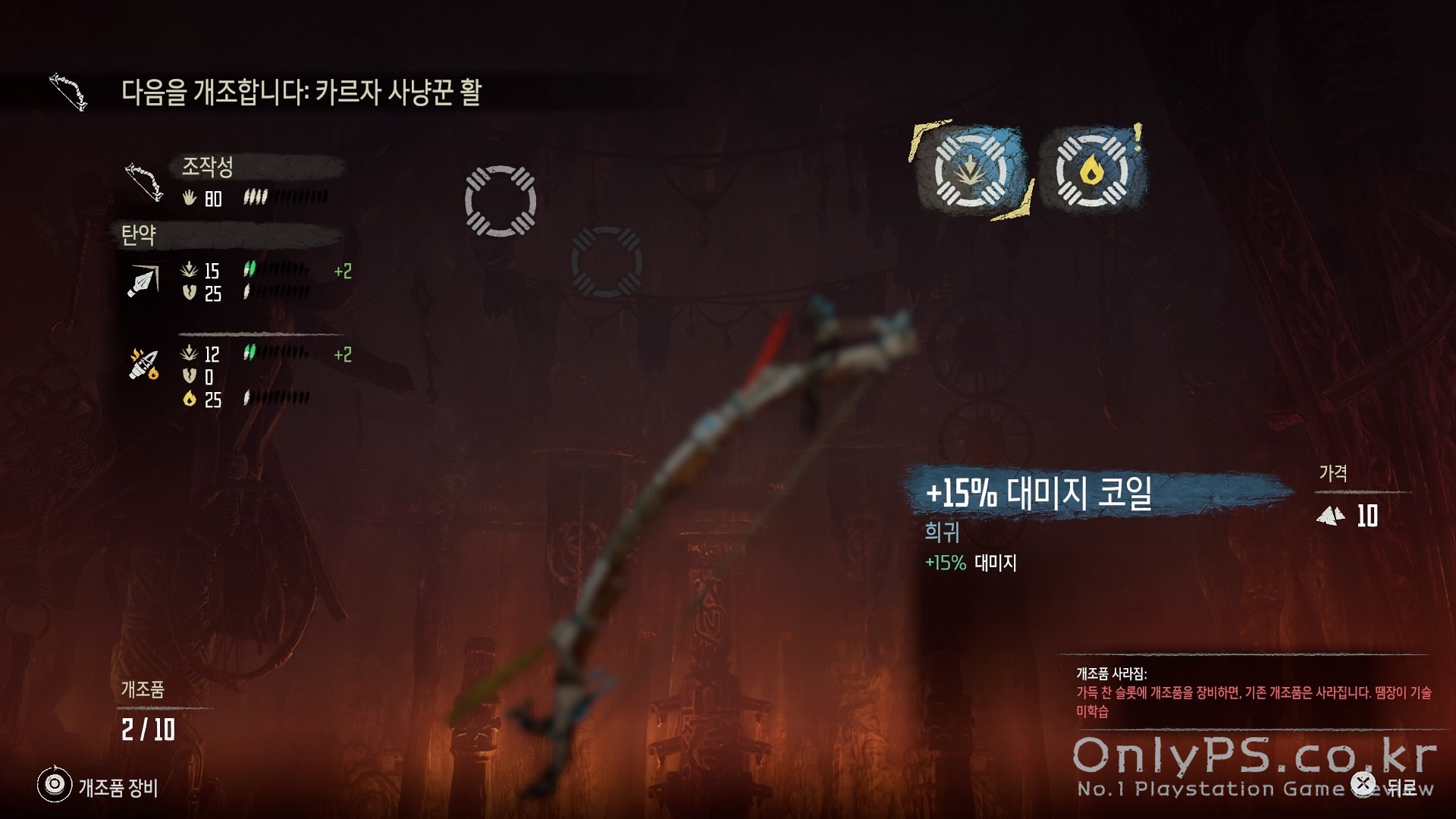This image is a detailed screenshot from a video game, featuring a rich, gradient background that transitions from almost black at the top through dark brown in the middle to a brighter brown at the bottom. Overlaying the background are various elements of the game's user interface, primarily presented in Korean, which can be seen in white text along the top and scattered throughout the image.

In the backdrop, vaguely discernible objects resemble totem poles or pillars, adding to the tribal aesthetic. Standing out in the middle is a mysterious silver rod-like object, curved and somewhat blurry, perhaps acting as a focal element or weapon in the game.

On the right side of the screen, there are circular badge-like symbols, each containing different icons, such as a plant and a flame, indicating different in-game stats or resources. Additionally, numbers and percentages, such as "15%", are displayed here, likely representing damage or other game metrics.

A scoreboard or inventory is also visible, displaying various numbers (e.g., 80, 15, 25, 12, 0, 25) paired with small icons, all contributing to the detailed game statistics. Notably, the bottom left corner shows "2 out of 10" with accompanying Korean text, perhaps referring to player status or some form of progress within the game.

At the very bottom of the image, a white watermark reads "only ps.co.kr," followed by "N.O.1 PlayStation game" and more Korean script, hinting at the game's origin or a promotional tagline. The interface elements, along with the layered gradient background and tribal-themed structures, give the screenshot a complex and immersive appearance.